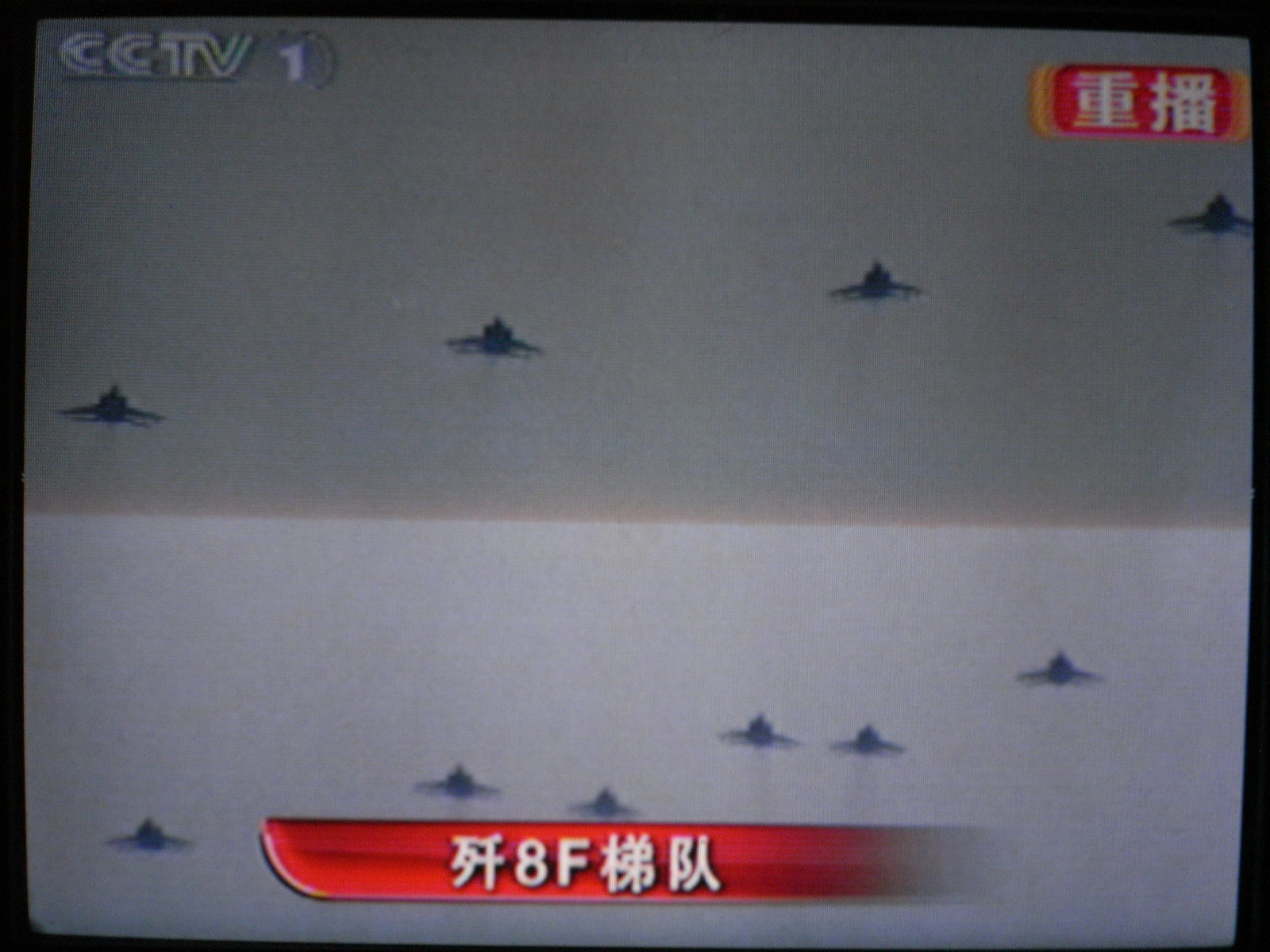The photograph, evidently taken of an older, cube-shaped TV screen, presents a somewhat blurry image dominated by a maritime and aerial scene. At the top left corner, the screen displays the text "CCTV1," while the top right features a red rectangle containing Chinese characters in white text. A similar red bar with white text, including three unreadable symbols followed by the number 8 and the letter F, spans the bottom of the screen. The main visual on the TV depicts a distant sea-to-sky horizon, with six distinct, black silhouette-like boats dotting the light blue ocean. Above, four dark, indistinct shapes, possibly fighter jets, glide through a predominantly gray sky. The overall atmosphere suggests a news broadcast capturing a scene from afar, with limited details due to the resolution and distance.